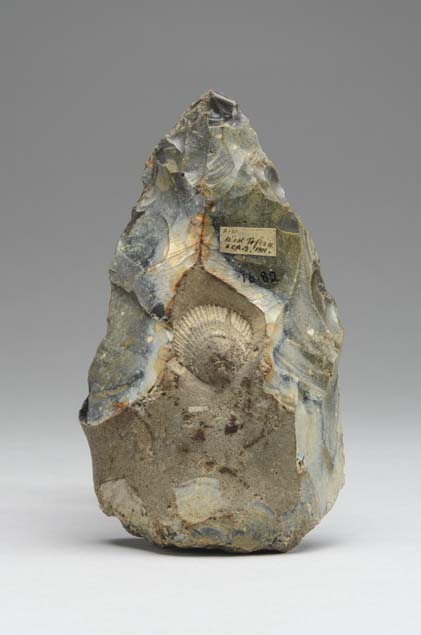This professional photograph features a triangular, almond-shaped rock that seems to be chiseled from the earth. Predominantly gray with slate, blue, and green hues, the rock is accentuated with white veins running through it. At the center, the rock showcases a fossil of a triangular-shaped seashell reminiscent of a clamshell, although the fossil appears weathered and asymmetrical. A piece of masking tape with some unreadable wording is affixed to the top right side of the rock, likely part of a documentation system for a collection. The image, set against a gray and white background, is high-resolution and meticulously captures the rock's intricate details and colors.